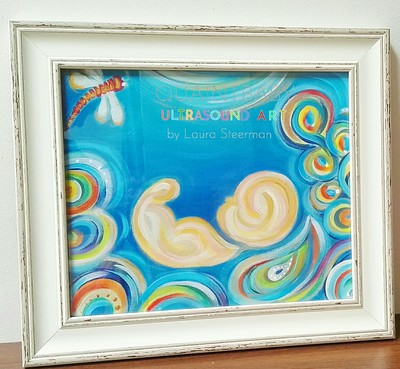The photograph displays a white, slightly distressed wooden photo frame sitting on a light brown wooden surface. Inside the frame is a piece of abstract artwork with a blue background, showcasing swirling colors such as red, orange, yellow, green, teal blue, and cream. Dominating the center of the artwork are two yellow blobs that form an abstract depiction of an unborn fetus, curled in what appears to be the fetal position. The swirls around the fetus shape include teardrop elements, and a small dragonfly is visible in the top left corner. At the center of the artwork, the words "ultrasound art" are written in multicolored letters, with the artist's name, Laura Stearman, appearing below in off-white text. The background behind the frame is a plain white wall.